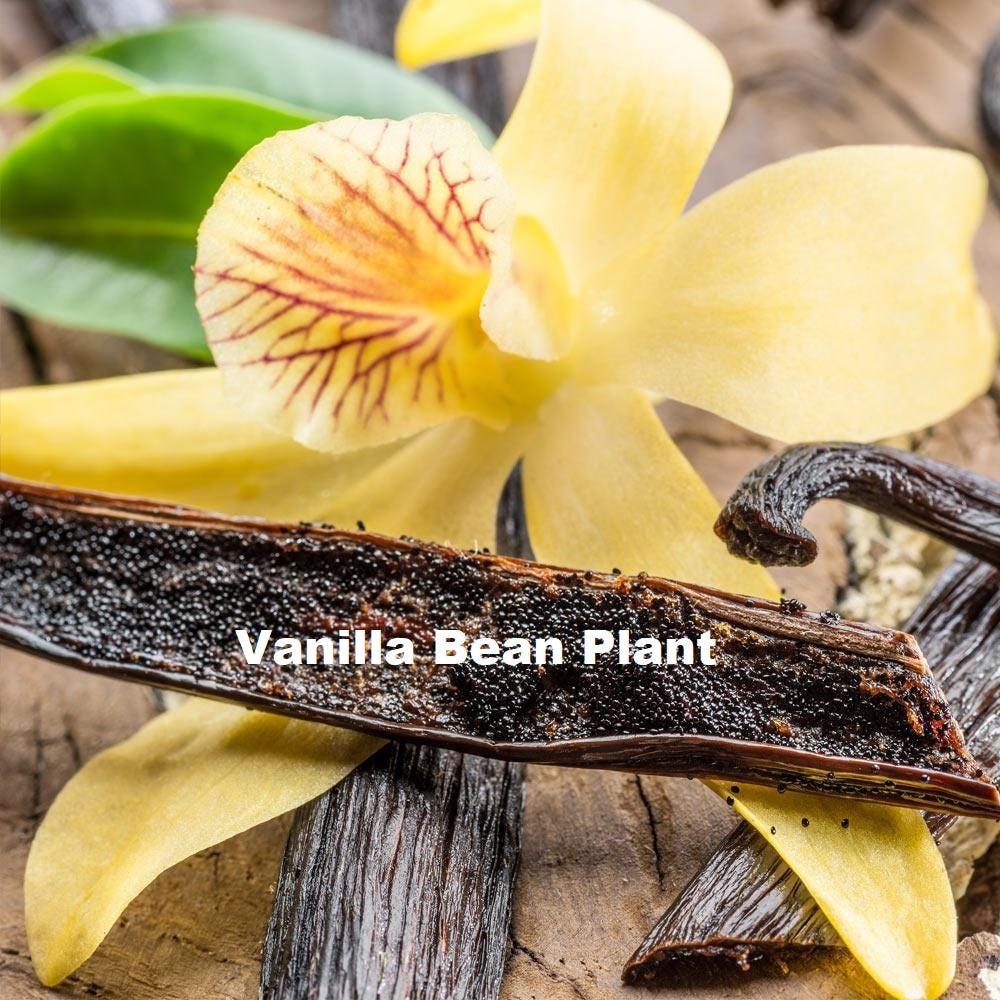The image depicts a vanilla bean plant in a detailed and striking composition. At the top, there is a bright yellow vanilla flower adorned with red vein-like markings on one of its petals, beautifully contrasting with the surrounding green leaves. The center of the image features an opened vanilla bean pod with its small, black seeds visible inside, showcasing the intricate details of the plant. The pod is labeled with white text reading "Vanilla Bean Plant." Additionally, there are two more unopened pods beside the opened one, all placed on a wooden table that grounds the scene. The background subtly highlights more green leaves, creating a lush backdrop. This image serves as an informative illustration of the vanilla bean plant, capturing its unique components and the process from flower to flavorful seeds.